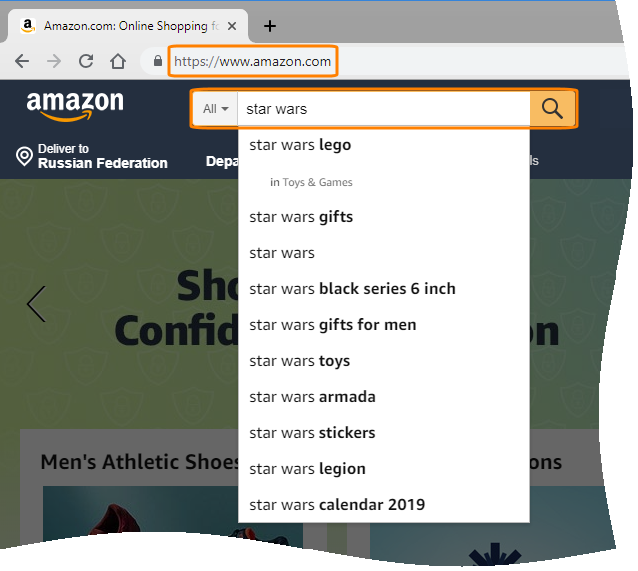This image is a modified screenshot featuring a search process on Amazon.com. The screenshot is vertically elongated with the top and left sides forming straight edges, while the right and bottom sides have a curved, scalloped design, indicating selective cropping.

The open browser tab clearly displays the Amazon homepage with the familiar Amazon logo positioned at the upper left corner of the screen. Below the logo, there is a notification indicating "Deliver to Russian Federation," suggesting that the user is browsing from Russia.

In the center of the image, the Amazon search bar, highlighted with an orange box, reveals that the user has entered the term "Star Wars." The website's URL is visible as "https://www.amazon.com." The search field auto-populates several product suggestions related to "Star Wars," including:

1. Star Wars Lego in Toys and Games
2. Star Wars Gifts
3. Star Wars
4. Star Wars Wax Series 6-inch
5. Star Wars Gifts for Men
6. Star Wars Toys
7. Star Wars Armada
8. Star Wars Stickers
9. Star Wars Legion
10. Star Wars Calendar 2019

The presence of the "Star Wars Calendar 2019" suggestion hints that the screenshot likely dates back to 2018 or 2019, making the image around three to four years old.